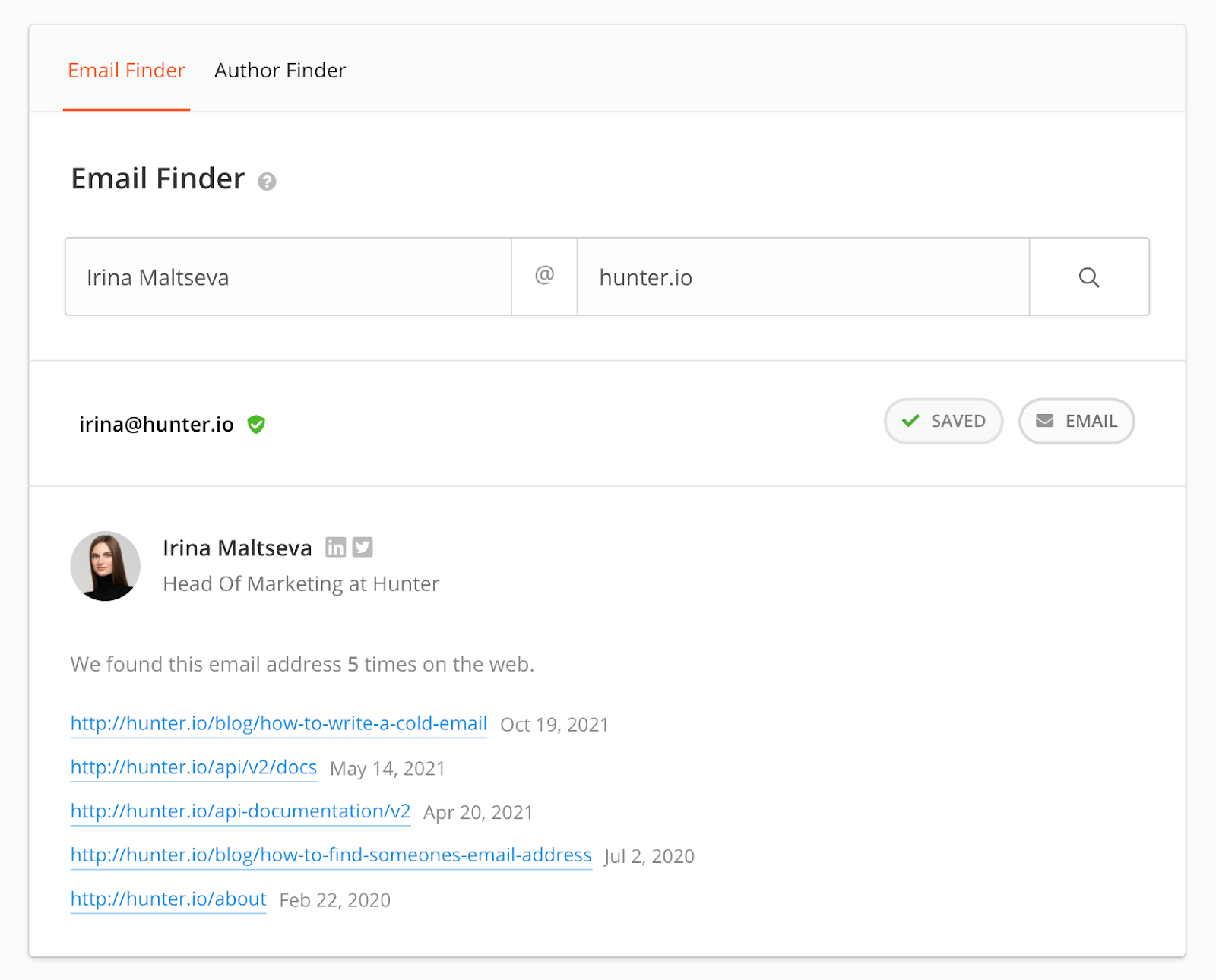The image depicts a detailed interface from Hunter.io, a tool used for finding email addresses. At the top, bold red text indicates functionalities like "Email Finder" and "Author Finder". The focus is on an entry for Irina Maltseva, with her email address, Irina@hunter.io, prominently displayed. Alongside her name, there are icons linking to her LinkedIn and Twitter profiles. Her role is noted as Head of Marketing at Hunter.io.

A green shield and an oval with a green checkmark signify verification or trustworthiness. Another oval labeled "Email" is present, along with a line separating sections of the interface. To the left, there's an image of Irina Maltseva.

Additional information includes a note that the email address has been found five times on the web, corroborated by several URLs and dates. These URLs point to resources and blogs related to email discovery and API usage:

1. [Hunter.io Blog: How to Write a Cold Email](http://hunter.io/blog/how-to-write-a-cold-email) - October 19, 2021
2. [Hunter.io API v2](http://hunter.io/api/v2) - Various dates including August and May 14, 2021
3. [Hunter.io Blog: How to Find Someone's Email Address](http://hunter.io/blog/how-to-find-someones-email-address) - July 2, 2020
4. [Hunter.io Blog](http://hunter.io/blog) - April 22, 2020

The background of the interface is white, bordered by gray edges, and interspaced with lines that may denote sections or links. This detailed summarization encompasses the relevant elements and structured information shown in the image.